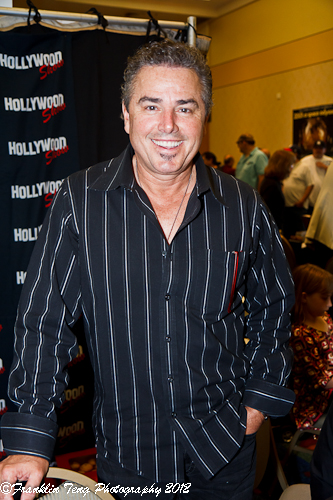In this image, a recognizable Caucasian male celebrity, reminiscent of a Brady Bunch star or Donny Osmond, is posing with a confident smile at a convention, possibly a meet-and-greet event. He features darker hair with some graying at the temples, thick manicured eyebrows, dark eyes, a broad smile, and a small patch of facial hair below his lower lip. His skin tone suggests he has recently been tanning. He is dressed in a navy blue button-down shirt with white vertical stripes and black pants, accessorized with a simple black cord necklace. In the photo, his left hand is casually placed in his pocket, while his right hand rests on the back of a chair. The background reveals a curtain adorned with the repeated phrase "Hollywood Show," indicative of the event setting. Notably, the image includes a visible watermark in the lower corner, crediting Franklin Tang Photography, circa 2012. A flash from the camera accentuates the subject, making him stand out against the surrounding crowd.